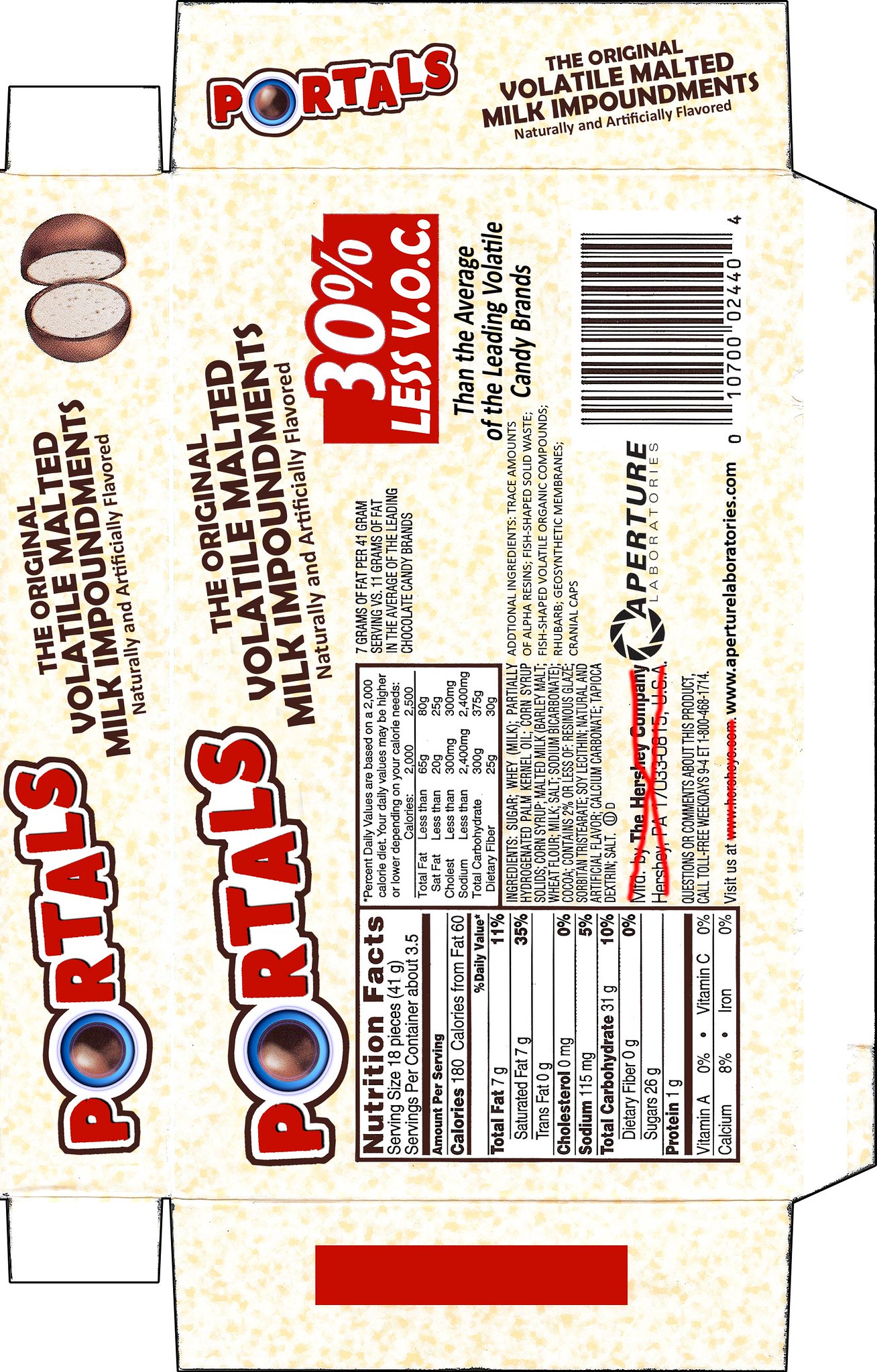This vertical photo showcases an individual serving box of candy laid flat on a surface. The box, titled "Portals," features the top side facing left and the bottom side facing right. The packaging is unfolded, revealing the edges that would typically be tucked in. The logo, "Portals," is prominently written in red and includes a silver ball with a blue border. This logo is positioned towards what would be the top side when the box is assembled, along with a larger section at the center of the image, which appears to be the back of the box. 

To the right of the logo, the text reads "The Original Volatile Malted Milk Impound Mints, Naturally and Artificially Flavored," printed vertically and tilted upwards to the right. A noticeable red rectangle near the corner states "30% Less VOC" in bold letters. A large barcode is situated at the bottom right side of the image. The far right edge of the image shows a white strip of the box, which would normally be tucked in and secured to form the complete box.